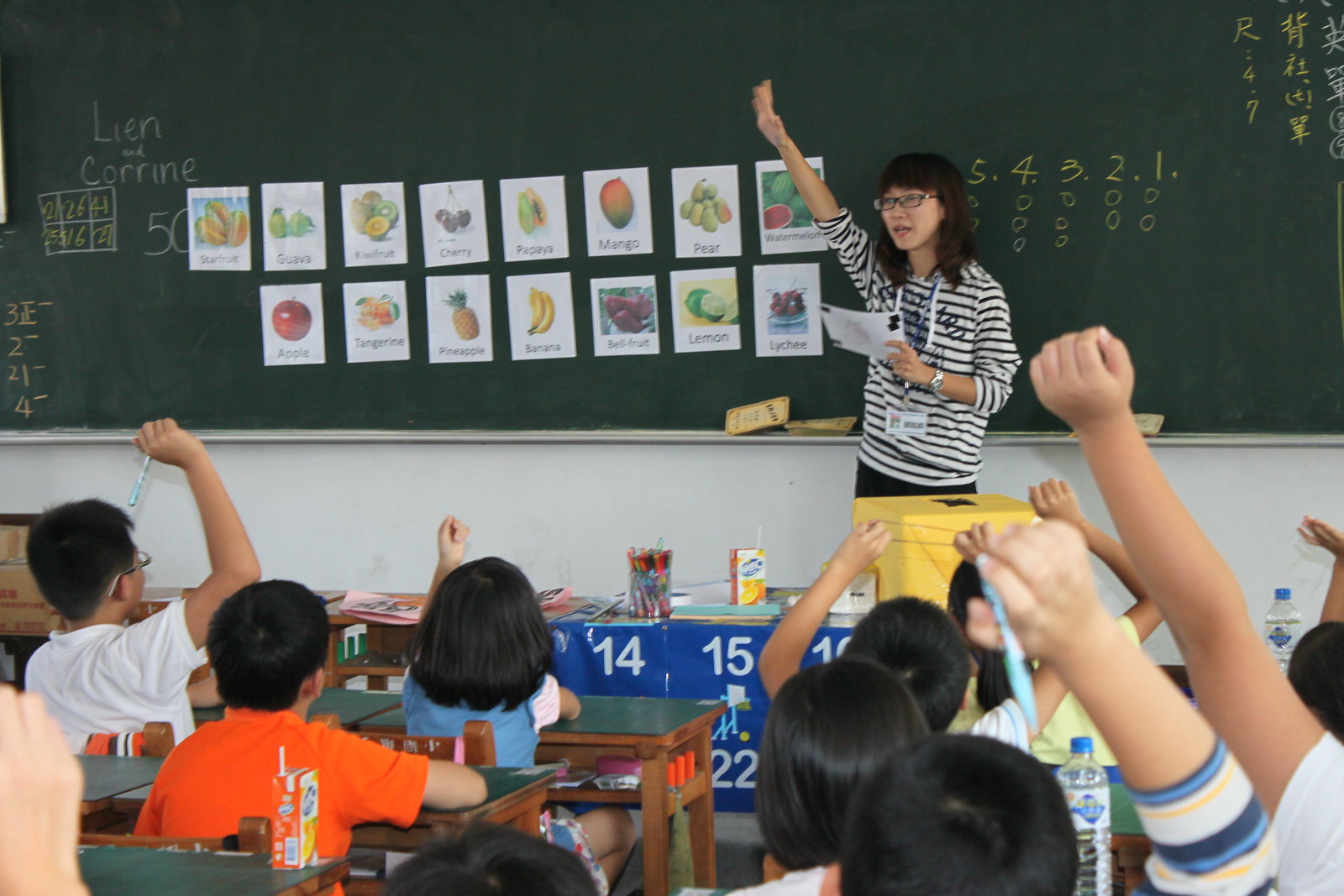This image depicts an elementary school classroom in Asia, likely China, based on the presence of Chinese writing on the green chalkboard in the background. The teacher, who appears to be Asian with long brown hair, eyeglasses, and a black and white pinstriped shirt, stands at the front of the room. She is raising her right hand, likely to encourage students to raise their hands if they know the answer. She holds a piece of paper in her left hand and wears a watch on her left arm along with a lanyard around her neck. Behind her, the green chalkboard is adorned with various pictures of fruits such as apple, banana, pineapple, mango, pear, lemon, and more, each labeled with their English names in white or yellow chalk, indicating an English lesson focused on fruit vocabulary.

Approximately 10 students are seated at desks with green tops and brown cubbies underneath. Many students have their hands raised, suggesting they are engaged and possibly responding to the teacher’s instructions. These children, all with dark hair, are facing the teacher, and a few of them are wearing eyeglasses. Additional numbers are taped to the front of the teacher's desk, enhancing the educational atmosphere of the scene.